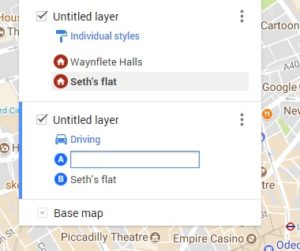In this image, the background features a detailed map covered by various labeled layers such as "Untitled Layer" and "Individual Styles." Prominently labeled areas include "Wind Fletch Halls" and "Sets Flats." Additionally, the image displays multiple instances of an "Untitled Layer" and elements associated with activities like "Driving." A search bar is visible towards the foreground, enhancing the utility of the interface. The color scheme prominently includes shades of red and blue, which accentuate the various map layers and elements, providing visual distinction within the graphic interface.